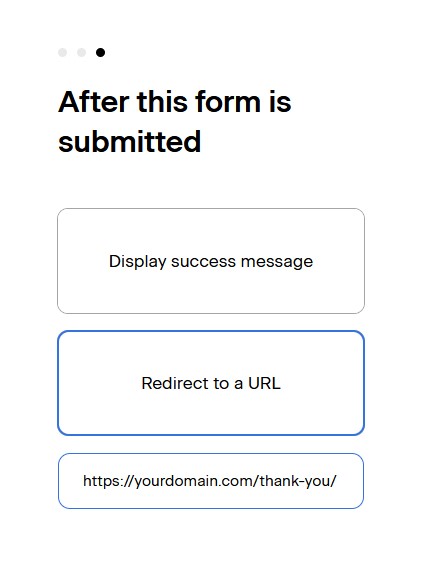In the upper right corner of the image, on the left-hand side, there are three circular buttons arranged side by side with a small gap between each. The first two buttons from the left are light gray, while the third button, furthest to the right, is black. Below this row of buttons, there is a space followed by text. In a larger font, it says, "After this form is," and on the next line, "submitted" is written in bold black font.

Beneath this text, there are two spaces, and then three boxes are displayed. The first box, located at the top, has a gray outline with a white center and contains the text "Display success message" in black font. The "D" in "Display" is capitalized. The second box features a blue outline with a white center and contains the text "Redirect to a URL" in black font. The third and final box has a thin light blue border and contains the URL "https://yourdomain.com/thank-you/" in black font.